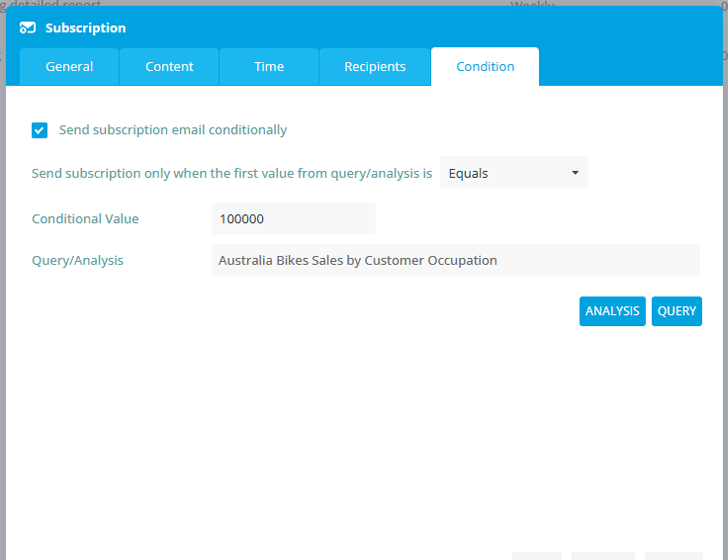This image displays a dialogue box from a computer application or website interface. The dialogue box features a blue header bar with a rectangular icon in the bottom left corner that contains a small clock. To the right of the icon, it boldly says "Subscription" in white text.

Below the header, there are several tabs that blend seamlessly with the background in a bluish hue. From left to right, the tabs are labeled "General," "Content," "Time," "Recipients," and "Condition," all in white text. The "Condition" tab is currently active, highlighted in a white button that leads to the main content window beneath it.

At the top of this main content area, there is a checkbox labeled in blue text, next to which it reads "Send Subscription Email Conditionally" in a greenish-blue color. Beneath this, another line of text reads "Send Subscription Only When the First Value from Query/Analysis is," followed by a dropdown box currently set to "Equals" in black text, accompanied by a small clock arrow on the right.

Further down, there is a line in a greenish color that says "Conditional Value." To the right of this text is a box displaying the number "100,000" in black text. Below this, once again in greenish text, it reads "Query/Analysis," with a search box to the right containing the selected entry "Australia Bike Sales by Customer Occupation."

At the bottom of the window, there are two blue buttons labeled "Analysis" and "Query," both with white text. The rest of the space along the bottom of the window is blank, filled with white space.